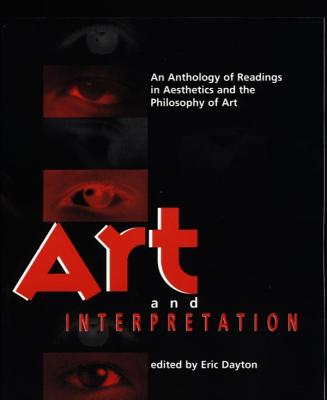The cover of the textbook "Art and Interpretation," edited by Eric Dayton, is predominantly black with striking red and white accents. "Art" is prominently featured in bold red at the top, followed by the small word "and" in white, and "Interpretation" in red at the bottom, albeit in a smaller font than "Art." The subtitle, printed in white, reads "An Anthology of Readings in Aesthetics and the Philosophy of Art." The background features a series of abstract, red-and-black shaded images of eyes— three along the left side and another at the bottom left. These eyes vary in design and seem to contribute to an enigmatic, artistic theme that complements the book's subject matter.